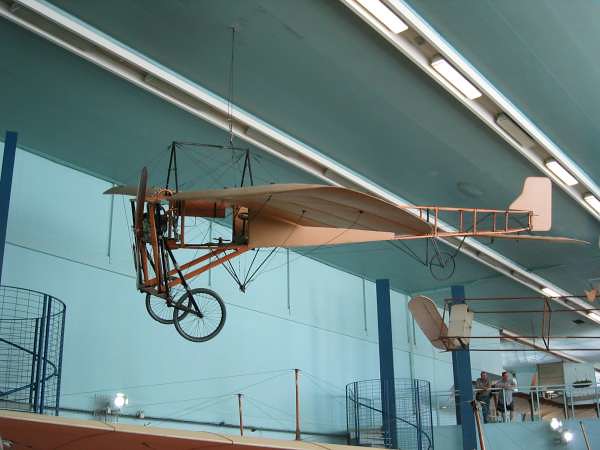This is a colored photograph taken indoors, likely inside an air and space museum. Prominently featured in the foreground is a large, old-fashioned model airplane hanging from the ceiling by thin wires. The airplane is reminiscent of the early aviation designs by Wilbur and Orville Wright, characterized by its wooden frame, wired spokes that resemble bicycle wheels, and simplistic construction with visible wings, a propeller, and a back tail. There are also a couple of men in the background, leaning against a metal railing or standing behind a metal walkway, observing the display. The ceiling and walls of the building are painted in a light blue color, and the ceiling is adorned with vertical lights arranged in a diagonal pattern. Additionally, behind the hanging airplane, there are other primitive aircraft or structures hanging in a similarly minimalist fashion, contributing to the museum's historic atmosphere. The setting includes circular metal areas with grid patterns, possibly spiral staircases or part of the museum's architecture, adding to the intricate detailing of the scene.